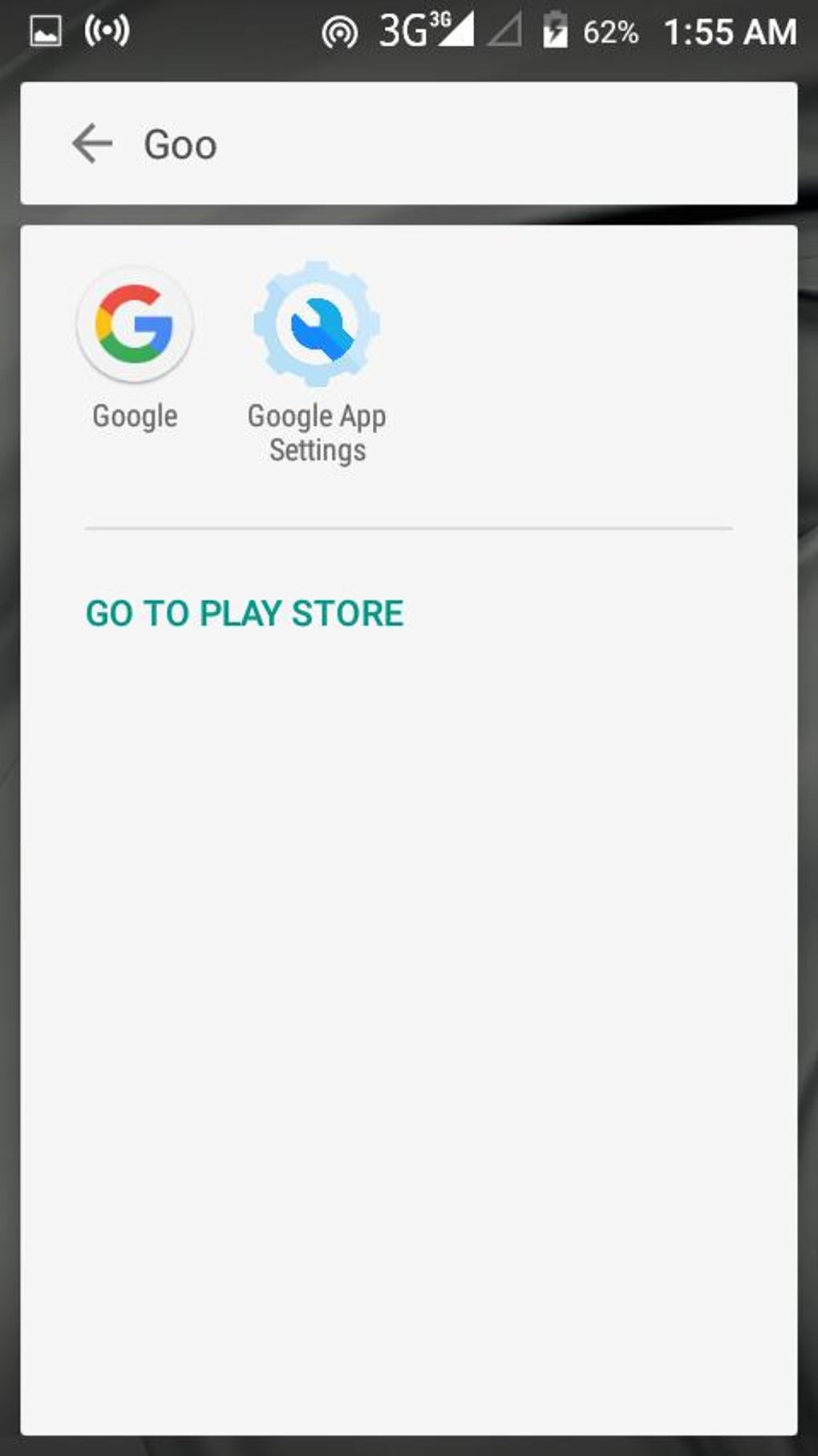This image is a screenshot captured on a mobile device's screen, showcasing a search interface. The background throughout the edges and along the top and bottom is charcoal black. In the upper left corner, there's a small white outline of a square containing icons that resemble little houses or mountains, indicative of some app or feature. Immediately to the right of it, a speaker indicator is visible. Toward the center of the top bar, there is a ring of circles, followed by white text displaying "3G36." Next to it, there's a signal bars indicator, which is followed by an empty Wi-Fi icon, indicating no Wi-Fi connection. Adjacent to these icons, a battery icon shows a 62% charge level. On the far right side of this top section, the time "1:55 AM" is displayed in white text.

Below this top bar, a white rectangle spans horizontally across the screen. Inside this rectangle, on the left side, there is a directional arrow pointing to the left, commonly used for navigation or stepping back in certain applications. Following the arrow is partial black text that reads "goo," likely part of a longer word or search query. 

Prominently centered beneath this is another large white rectangle occupying a significant portion of the screenshot. In the upper left corner of this rectangle is the iconic multicolored Google "G" logo, composed of red, yellow, green, and blue segments. Directly below this logo, the word "Google" is printed in black text, signifying the main Google app or search engine. To the right of this logo and text, there is a settings icon for the Google app, represented by a light blue gear with a darker blue wrench head in the center. Underneath this gear icon, the text "Google app settings" is printed, indicating access to the app's settings.

There is a thin light gray line running horizontally beneath this section. At the bottom of the screenshot, there is a text in greenish-blue color that reads "Go to Play Store," suggesting an option or link to navigate to the Google Play Store for downloading additional apps or content.